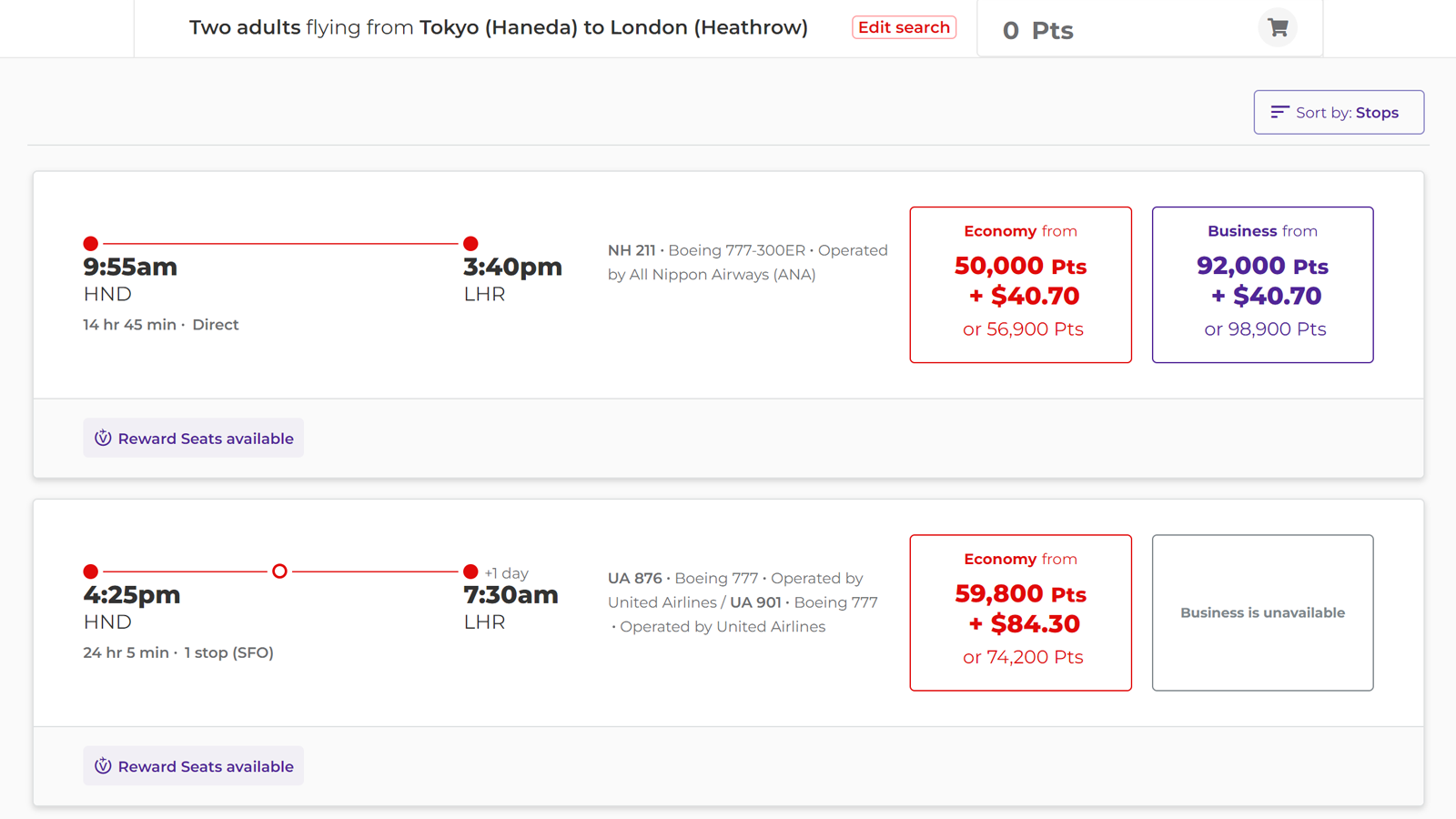In the image, we see a screenshot of a travel booking website set against a slightly grayish background. At the top, in black text, the details are displayed as follows: "Two adults flying from Tokyo Haneda to London Heathrow." To the right of this information, there is an option to edit the search, accompanied by a notation indicating "zero points." Further to the right, there is a shopping cart symbol.

Below this top section, there are two primary white boxes containing flight details. In the first box, the departure is from Haneda Airport at 9:55 a.m., arriving at London Heathrow at 3:40 p.m. On the right side of this box, there are various fare options: 
- Economy: 50,000 points plus $40.70 or 56,900 points.
- Business: 92,000 points plus $40.70 or 98,000 points.

Additionally, a note on the left states that reward seats are available.

In the second box, there is another flight option departing from Haneda at 4:25 p.m. and arriving at London Heathrow at 7:30 a.m. The fare options in this section are as follows:
- Business class is marked as unavailable.
- Economy: 59,800 points plus $84.30 or 74,200 points.

Overall, the image provides detailed information on flight availability and fare options for a journey from Tokyo Haneda to London Heathrow.